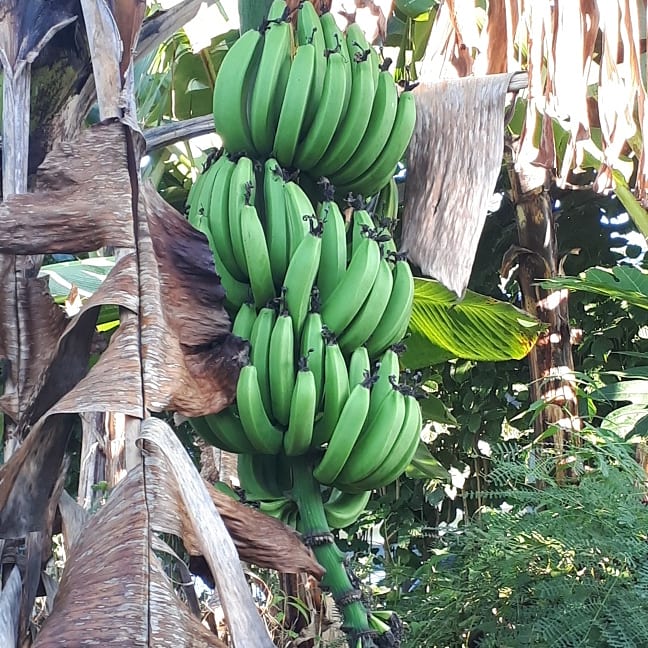This vibrant outdoor photograph depicts a cluster of unripe, vibrant green bananas hanging from a thick, bamboo-like stem in what appears to be a deep jungle setting. The bananas are organized in three distinct rows, each row comprising hefty and long bananas. Interestingly, these bananas are oriented facing upwards. Surrounding the main banana cluster are various large tropical plants, including a significant plant with sizeable, cocoa-brown leaves, giving the scene an exotic backdrop. In the lower right corner, greenish fern-like foliage is visible, adding texture to the scene. Dappled sunlight filters through the upper right of the image, illuminating brown and white plant matter and enhancing the rich, tropical ambiance. The thick stem of the banana plant and the lush, green and brown foliage suggest a hearty, thriving jungle environment.